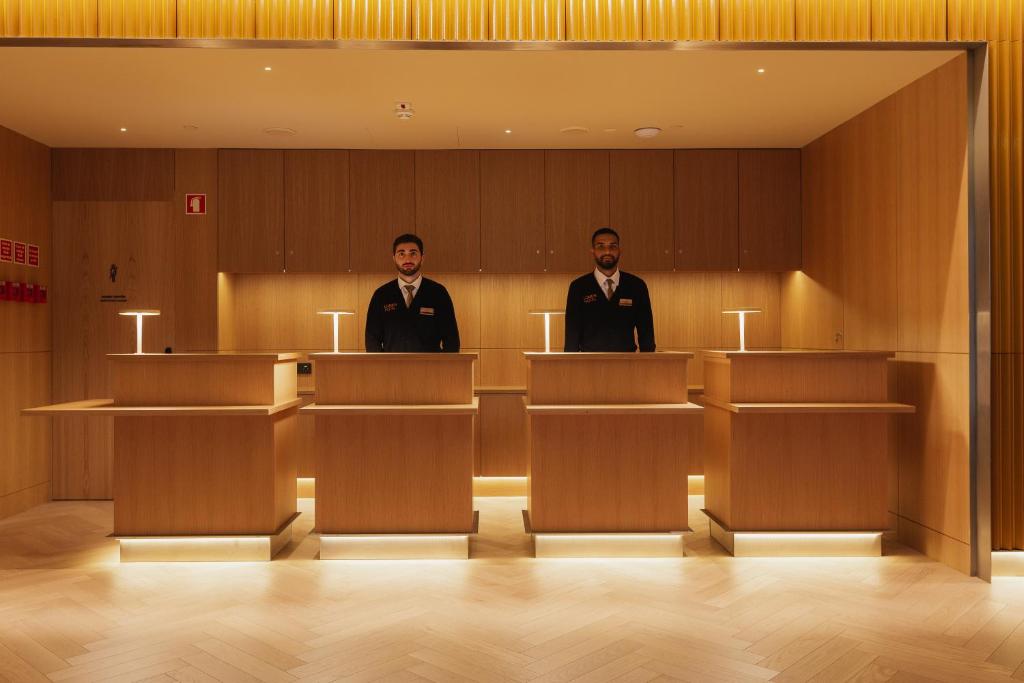In this image, we see two men standing in what appears to be a hotel lobby, likely serving as concierges or receptionists. Both men are dressed in black sweaters over white collared shirts paired with brown ties, and they wear nameplates on their right chest. The man on the left is light-skinned with a brown beard and short brown hair, while the man on the right has a darker complexion, possibly African American, and also sports a beard with short brown hair. They are standing behind brown wooden podiums or counters.

The room is richly decorated with brown wood paneling on the walls, wood floors, and wood ceilings, creating a warm, rustic ambiance. Illuminating the setting, there are discreet lights embedded in the base of the podiums and overhead, providing a soft, welcoming glow. To the left, an emergency exit door can be seen, along with red warning signs, enhancing the safety features of the area. The overall scene exudes a professional yet cozy atmosphere within this hotel lobby.